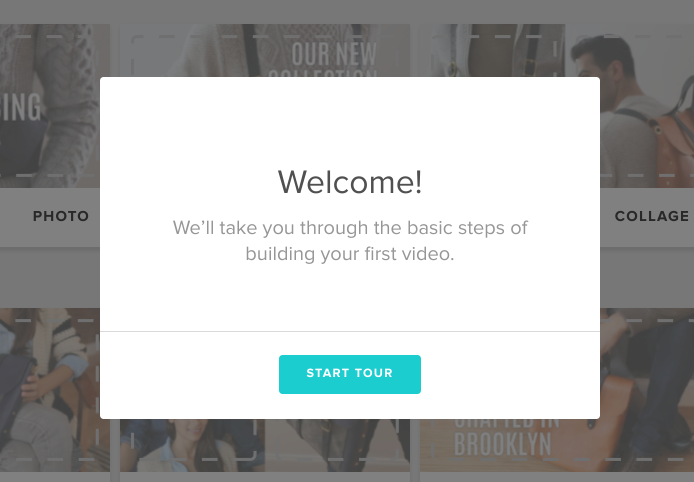The image features a prominent white pop-up box at the center that reads "Welcome!" in large letters. Below this in gray text, it states, "We'll take you through the basic steps of building your first video," with a blue "Start Tour" button beneath it. The website behind the pop-up is partially visible and consists of three rows of images, each bordered with dotted lines reminiscent of a cut-out coupon pattern.

In the top row:

- The first image is labeled "Photo" and shows part of a person wearing a sweater, with only their midsection and arm visible. The text "ing" is partially visible, but the full word is obscured.
- The second image is titled "Our New Collection," although only "Our New" and part of "Collection" is visible. It displays a person in a white sweater.
- The third image is labeled "Collage" and shows a man with short hair, turned slightly to his left, wearing a leather backpack with a black strap.

In the second row:

- The first two images show a person with crossed legs holding what looks like a laptop bag in their left hand, another person smiling directly at the camera, and a series of dresses.
- The last image depicts a hand picking up a leather briefcase with black handles. The text on this image seems to say "Crafted in Brooklyn," but part of the phrase is cut off.

Every image in the rows is framed by the same dotted borders, maintaining a cohesive design throughout the website preview.